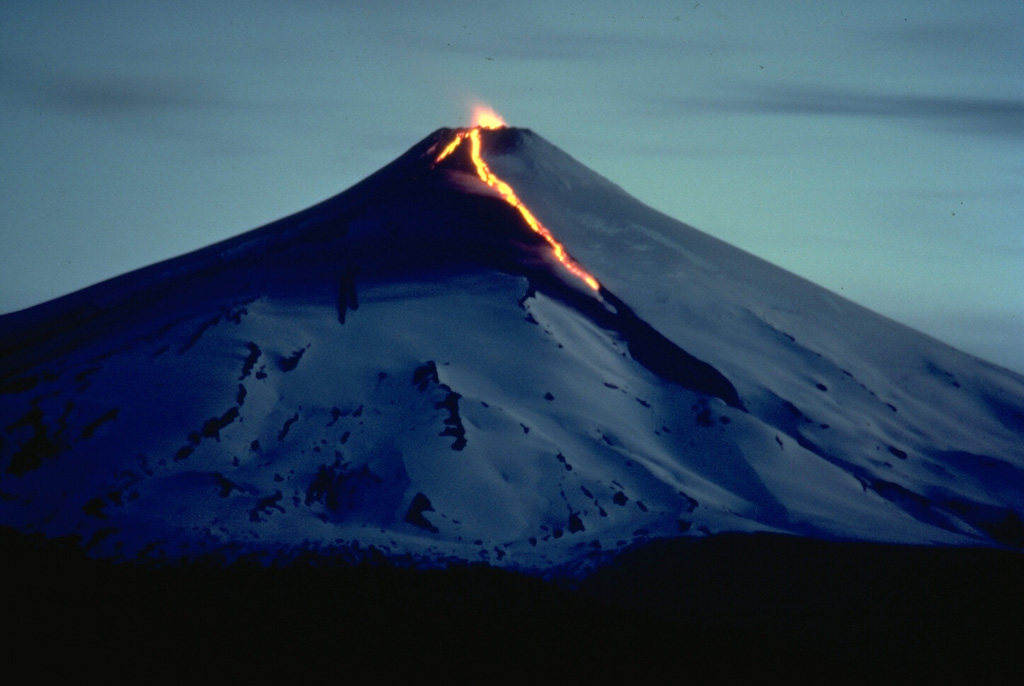The photograph has a nostalgic, grainy feel, suggesting it might have been taken with an older or less sophisticated camera, likely using film. The image captures a dusky or twilight scene, with the light fading but not entirely gone, casting a dark blue-gray ambiance. The very bottom of the photo, possibly treetops or the ground, is enveloped in darkness, obscuring exact details.

Dominating the center of the image is a volcano, which appears to be modestly erupting. There's no large plume of smoke, but two distinct streams of glowing, molten lava, one longer and more prominent while the other is just beginning. The volcano itself is mostly covered in a light grayish snow, with some darker rocky outcrops piercing through, particularly noticeable on the left side. This contrasts starkly with the vibrant yellow-orange of the lava. The overall setting evokes a dramatic and serene nocturnal landscape, with the natural phenomenon of an eruption highlighted against the tranquil, almost ethereal twilight sky.